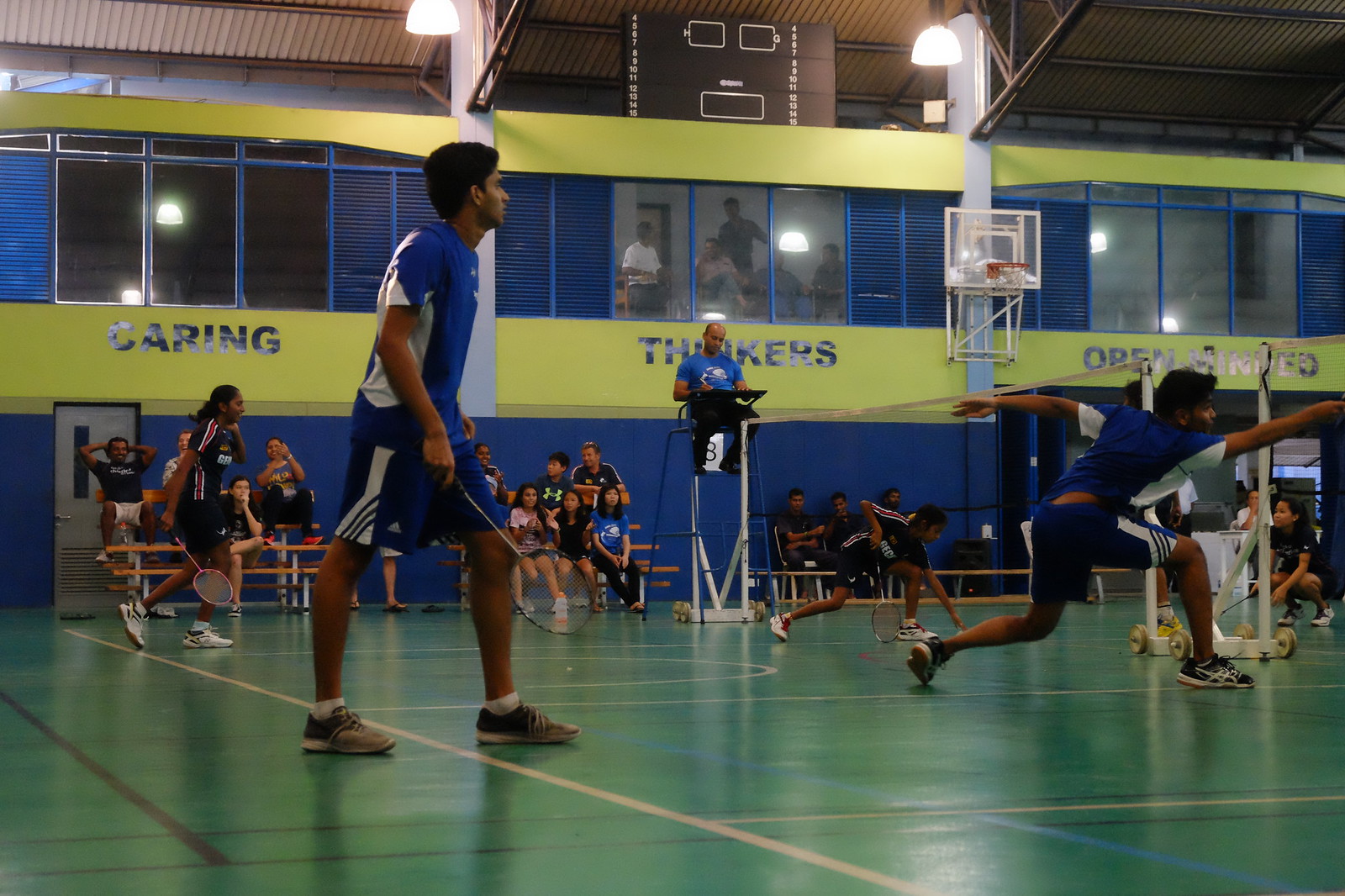This color photograph captures an intense badminton game in a vibrant gymnasium, distinguished by its green floor and walls painted in a combination of blue and yellow with motivational slogans. The photograph is taken from the corner edge of the court, focusing on a doubles match in the foreground. Both teams are wearing coordinated blue and white uniforms, with the players holding their rackets in their right hands. The player nearest to the net is lunging forward, having just hit the shuttlecock. Behind them, two players in the back are attentively observing the game's progress. 

In the background, a referee in blue and white attire is seated on a high podium, overseeing the match, possibly referencing information from a computer. Further behind, there's another visible match featuring women's doubles, where the participants also sport uniforms but with dark blue and red accents. Spectators are present, some seated on wooden bleachers along the blue wall and others standing, engaging with the unfolding matches. A basketball net, pulled to the side, hints at the multi-functional use of the gymnasium. Above the action, windows provide a glimpse of additional spectators and passages featuring slogans that promote positive values. A gray door in the lower left corner likely serves as an exit, completing the detailed scene of this lively badminton game.